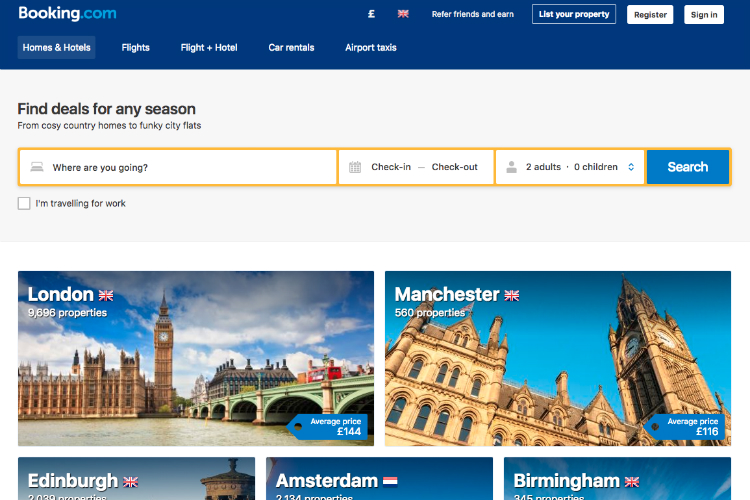This is a detailed description of the Booking.com website homepage. The website features a prominent blue navigation bar at the top with the “booking” text in white and “.com” in light blue. To the right of the logo are icons for currency (a pound symbol), a UK flag for language selection, links to refer friends and earn rewards, options for property owners to register with the site, and sign-in functionality.

Below the navigation bar, there are tabs for different services such as "Homes & Hotels," "Flights," "Flight & Hotel," "Car Rentals," and "Airport Taxis." Underneath these tabs, there is a grey box with promotional text that reads "Find deals for any season from cozy country homes to funky city flats."

Highlighted in yellow, boxes prompt the user to enter their destination, check-in and check-out dates, and specify the number of adults and children traveling. There is an additional checkbox option labeled "I'm traveling for work." 

Below the search section, the website displays featured destinations including London, Manchester, Edinburgh, Amsterdam, and Birmingham, along with the number of available properties and their price ranges.